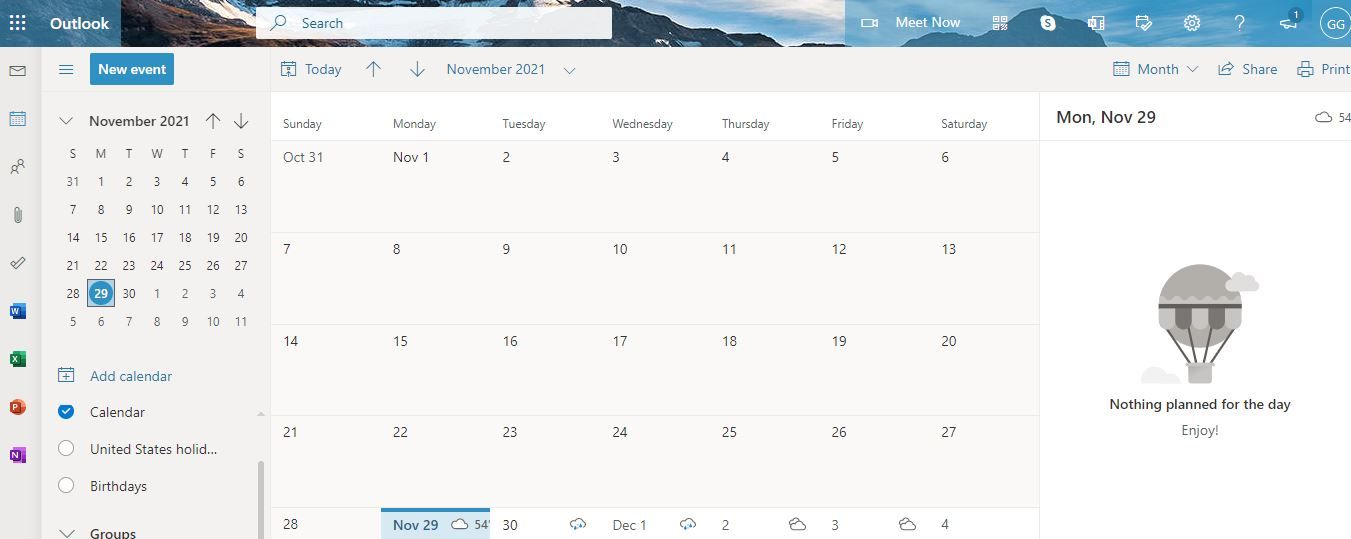The image is a detailed screenshot of an Outlook calendar interface. At the top, a horizontal bar displays the 'Outlook' logo on the left. The background features a scenic landscape of mountains. Adjacent to the logo is a search bar, followed by various clickable icons—'Meet Now,' a Windows logo, an 'S' which likely represents Spotify, a text icon, settings, and a help icon.

On the left sidebar, there are options for 'Mail,' 'People,' 'Word,' 'Excel,' and additional links. Below this, a condensed calendar view is set to November 2021, with the 29th of November highlighted. Directly below, there's an option to 'Add Calendar,' followed by selectable categories such as 'Calendar,' 'United States,' 'Birthdays,' and 'Groups.'

The main section of the screen shows a monthly calendar for November 2021, but no events are listed. To the right, for the day view of Monday, November 29th, there is an image of a hot air balloon with the message, "Nothing planned for the day. Enjoy."